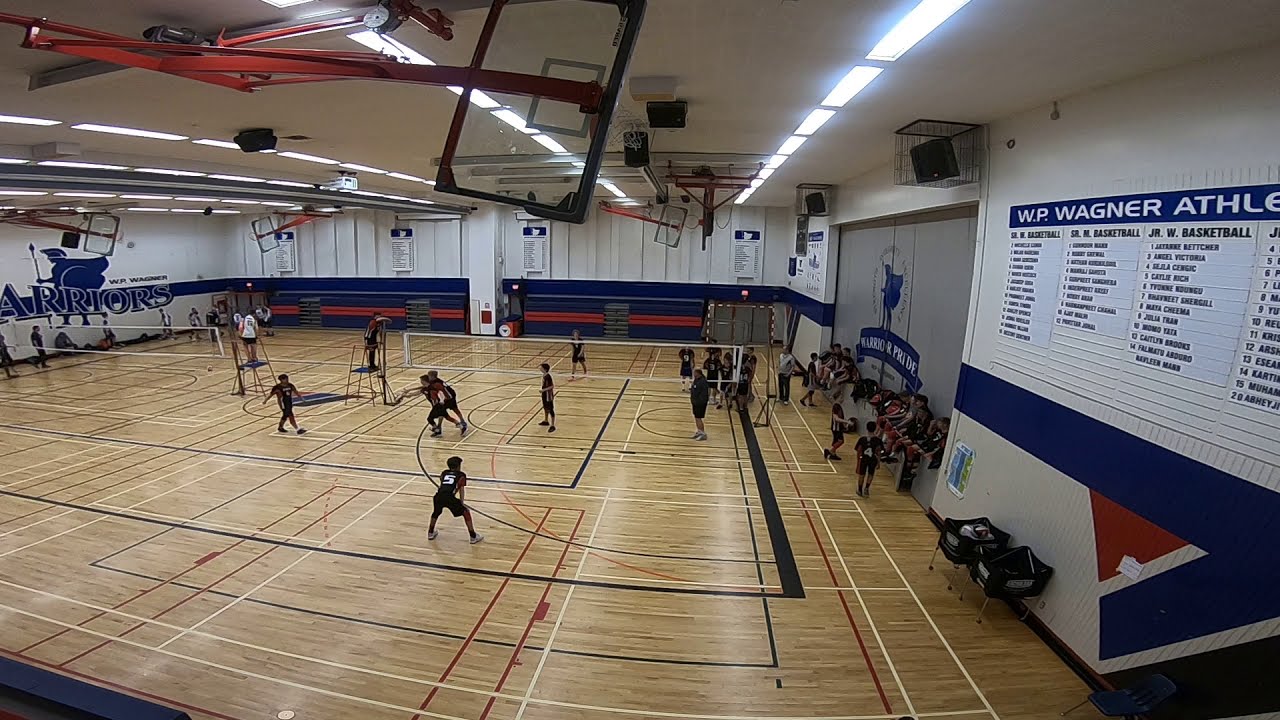This image captures an indoor basketball court that has been repurposed into a volleyball court. The gym features two volleyball nets set up across the court, indicating the possibility of simultaneous games. Basketball hoops are retracted upwards, secured by red and white scaffolding against the white ceiling. Rows of white fluorescent lights illuminate the spacious gym.

The walls are predominantly white, accented with blue and red padding along the far wall. Mounted speakers, protected by cages, are visible on the ceiling. On the far left wall, there's a mural of an ancient warrior, with the word "Warriors" painted above it, aligning with the school's theme. 

An active volleyball game is taking place on the right side of the court, with players in numbered jerseys, including a noticeable player wearing a dark jersey with a number five in white. A prominent sign on the right wall reads "WP Wagner Athletics," accompanied by a list of names, likely the school's athletes. The gym’s decor prominently features white, blue, and red colors, reinforcing the school spirit and identity.